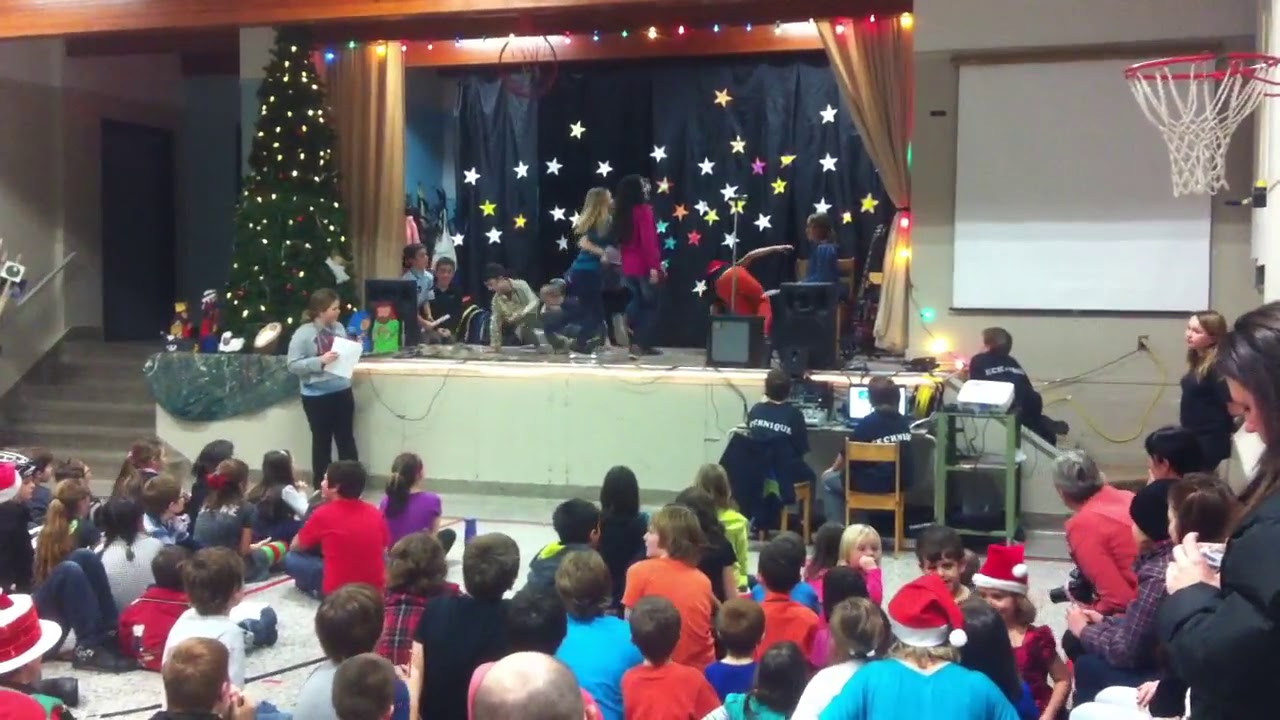This detailed photograph captures a festive Christmas pageant taking place in a school gymnasium. The focal point is a raised stage positioned towards the upper center of the image, adorned with a backdrop of a dark black curtain littered with bright stars, enhancing the holiday theme. On the stage, children dressed in everyday attire are engaged in both sitting and standing positions, depicting their performance.

Flanking the stage on the left is a lit Christmas tree surrounded by festive packages and ornaments. Adjacent to the tree, an open stairwell with a railing leads down into the auditorium, marked by a white wall with an open doorway at its summit. On the right side of the stage, a pull-down projector screen hangs from the ceiling, with a basketball backboard and hoop visible at the upper right edge, emphasizing that the setting is indeed a gymnasium.

In the foreground, students sit on the floor attentively watching the performance. Standing in front of the stage, beneath the Christmas tree, is an adult woman wearing a gray long-sleeve sweater and black pants, holding a microphone and reading from a paper, possibly narrating or directing the event. Additionally, there is an area to the lower right of the image, near the audience, featuring a desk, a cart, and some chairs with computers, suggesting assistance with the production.

The vibrant scene is imbued with a spectrum of colors including red, orange, yellow, green, blue, purple, pink, coral, black, white, silver, gray, beige, brown, dark blue, turquoise, aqua blue, and magenta, undoubtedly enhancing the joyous atmosphere of the Christmas pageant.